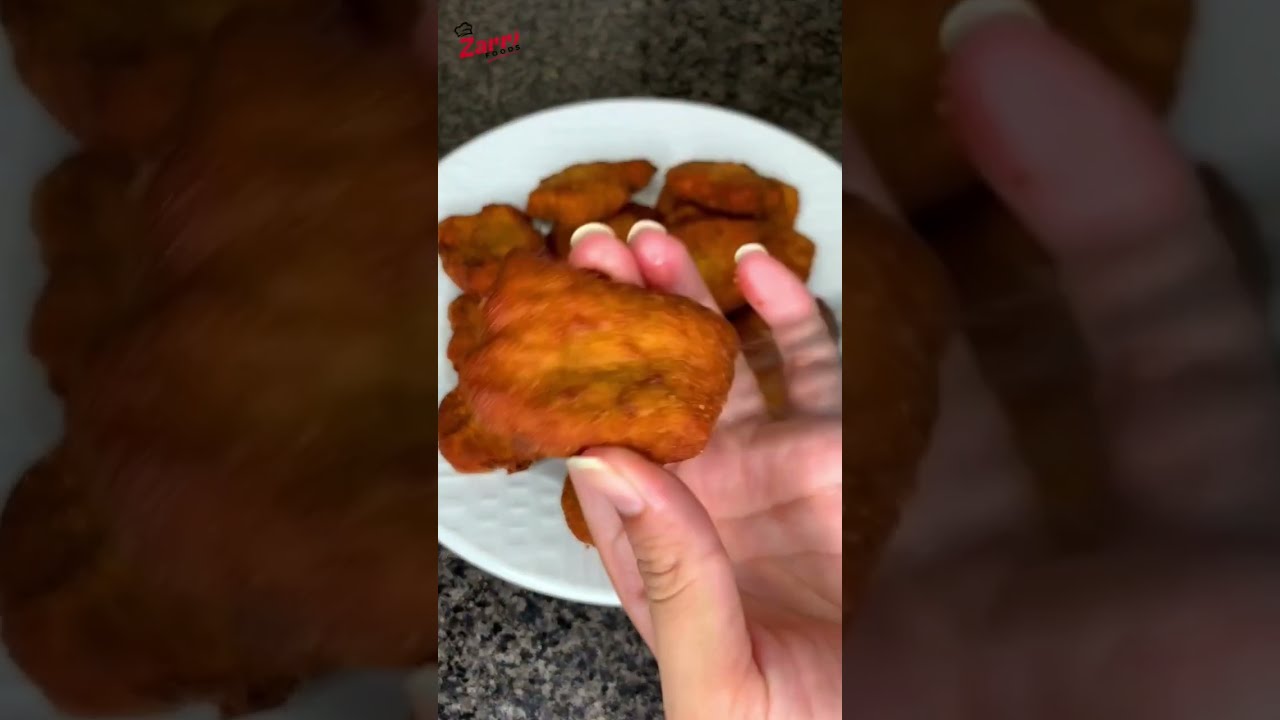This image is a screencap from a social media video characterized by its longer vertical edges and shorter top and bottom edges, indicating a mobile-friendly format. The central part of the image features a detailed view of a woman's hand with long white fingernails, palm up, delicately gripping a dark, crispy golden brown deep-fried item—likely a chicken nugget or tender—between her thumb and middle finger. The woman's hand is set against a white round porcelain plate laden with more similarly breaded and jagged-edged chicken nuggets, which rest on a marbled countertop in tones of white, gray, and black. The video has been zoomed in around the center, creating black-filtered sections on the left and right sides of the image to fit the screen. A red watermark with the letters "Z-A-R-R" is prominently displayed at the top left corner, adding a branded touch to the scene. The overall composition highlights the delicious, appetizing texture and color of the food, complemented by the clean, modern setting.